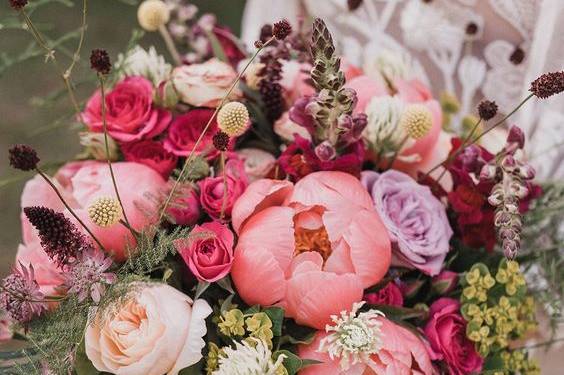This close-up aerial photograph showcases an exquisite, tightly bunched bouquet of flowers, potentially intended for a party, event, or wedding. The bouquet predominantly features various shades of pink, from light to medium and dark, including maroons, with numerous small and large pink roses. Interspersed among the roses are carnations, light lavender blooms, and splashes of yellow and white. Some flowers, particularly a large bloom at the center, are partially closed, revealing delicate openings. Adding to the bouquet's lush appearance are stems with small brownish seed heads, deep purple accents, and a mix of soft greenery and fillers. In the blurred background, an ornate white object with decorative designs subtly enhances the bouquet's elegant presentation. The varying heights and layers of the flowers create a full, dimensional arrangement, making the bouquet appear rich and vibrant.